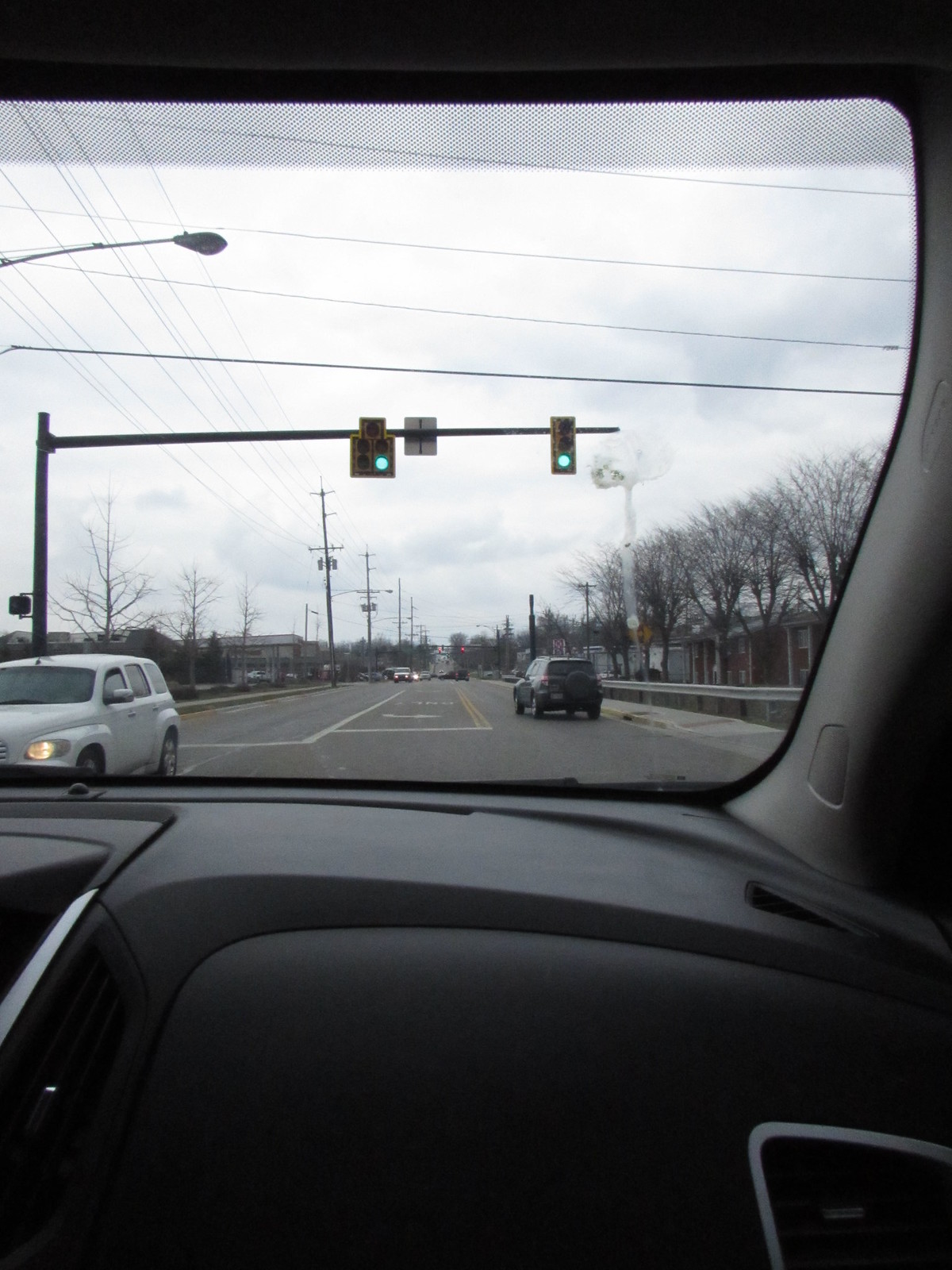This photograph captures a moment from the passenger seat of a small car, positioned in the left turn lane at an intersection. The vehicle features a right-hand drive configuration, typical of countries like the UK or Japan. In the foreground, a white, compact station wagon passes by, while a blue car ahead proceeds through the green traffic light. Guardrails flank both sides of the road, providing a sense of safety and structure.

On the left, buildings stretch into the distance, juxtaposed against a row of uniformly shaped trees lining the right side of the street. The vista extends to reveal more vehicles approaching from the opposite direction. The entire scene is enveloped in a muted, overcast ambiance, characterized by gray skies and a lack of vivid color, conveying a quiet, uneventful atmosphere.